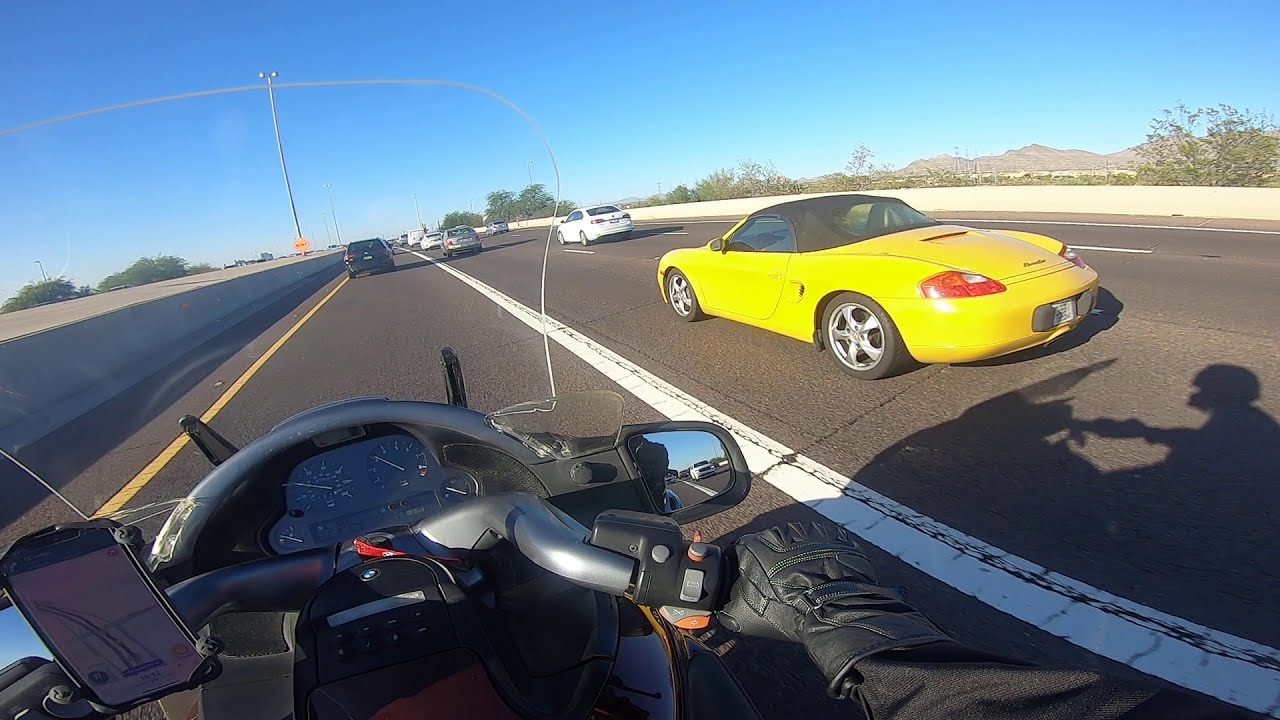The image captures a dynamic scene from the perspective of a motorcyclist navigating a multi-lane highway on a bright, sunny day. The motorcyclist's gauntleted hands grip the handlebars, with a visible instrument panel and a GPS providing directions. To the right, a bright yellow Porsche convertible with a black top, situated in the adjacent lane, stands out prominently. Slightly ahead of the motorcycle is the shadow it casts on the road. Just ahead of the Porsche, a white sedan cruises along, followed by a silver sedan and other vehicles extending further down the highway. To the left of the motorcyclist, a yellow line separates the lane from a concrete barrier. Further details reveal a power pole in the upper left corner, additional cement barriers on both sides of the highway, scattered shrubbery, and distant hills under a pastel blue, hazy sky.